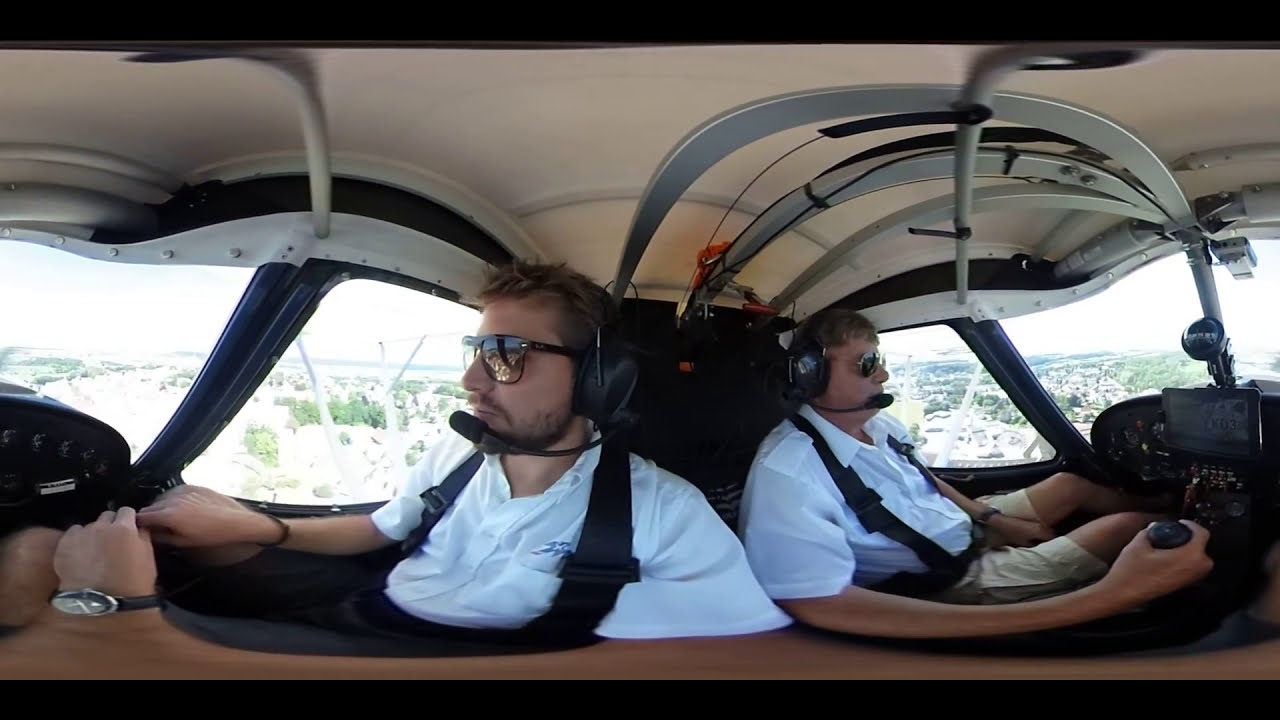This image captures the interior of a small airplane in flight, emphasizing the focused atmosphere of the cockpit. The compact plane has room for only two individuals, who are centrally positioned in the frame. Both men are adorned in white button-up shirts, with the person on the left featuring a blue logo on the chest. They also sport black wristwatches and headsets with large microphones. Their accessories include sunglasses with black reflective lenses— the left person wearing black-rimmed ones, and the right person, silver-rimmed. The one on the right adds a casual touch with khaki shorts. The cockpit's interior presents a white roof and predominantly black fixtures, with a backdrop view of an urban landscape through the windows. The left individual is actively engaging with the dials, while the right person, who appears slightly older, is maneuvering a black stick, likely the control column, emphasizing their roles as pilots. Their light brown hair and symmetrical seating contribute to the organized and professional vibe of the photograph.